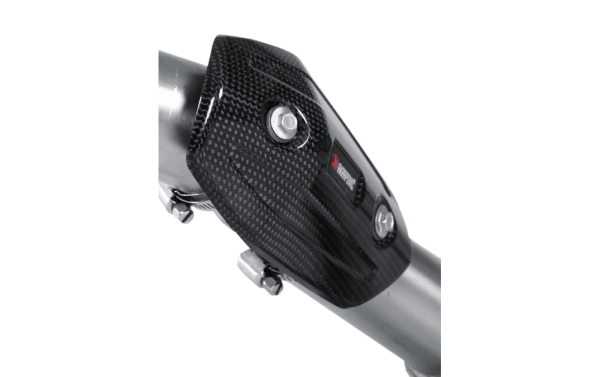This color photograph, in portrait orientation, features a very close-up view of two thick, smooth, silver metal pipes with a glossy, space-gray finish. The pipes, possibly handlebars of a bicycle, intersect in the center of the frame and are connected by a black rectangular plate with a waffle pattern on the left and a smooth right side. The black connector, which might be made of plastic or metal, is secured onto the pipes by collar screws. Additionally, there are two horizontal bolts or screws attached to its top and bottom on the left and right sides, respectively. Between these screws, there is a flat, smooth oval logo featuring a red symbol that resembles a peace sign, followed by illegible white text. The entire background of the image is pitch black, highlighting the reflective surface of the metal pipes and the contrasting textures of the black plate. The lighting accentuates the glossy finish of the pipes, adding to the detailed realism of the photograph.